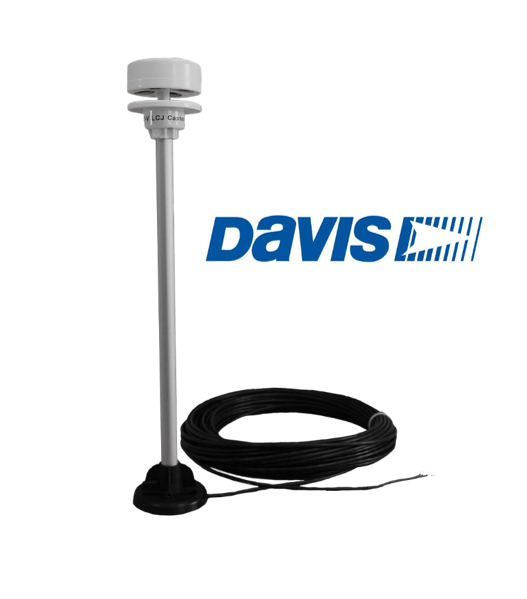The image depicts a light stand or signal device set against a white background, likely intended for advertisement or an online shopping platform. The main focus of the device is a tall silver pole approximately 2 to 3 feet in length. At the top of the pole, there is a circular disk that features four holes on its underside, and beneath it, another disk with a tapered base. The upper sections of these components are white, with a possible indication of black writing on them.

The pole extends down to a black base, which appears to be made of plastic or rubber. From this base, a long black cord emerges, coiling tightly into a neat circle before extending off to the right side of the image. The coiled cable and base suggest the device is designed to be plugged in, although it is not illuminated in the image.

Positioned centrally and slightly to the right is the text "Davis" in blue, accompanied by a logo consisting of white arrows pointing to the right, intersecting a background of hash-marked blue lines. This imagery implies the device may be used in industrial or store settings and provides a clear and informative preview for potential buyers.